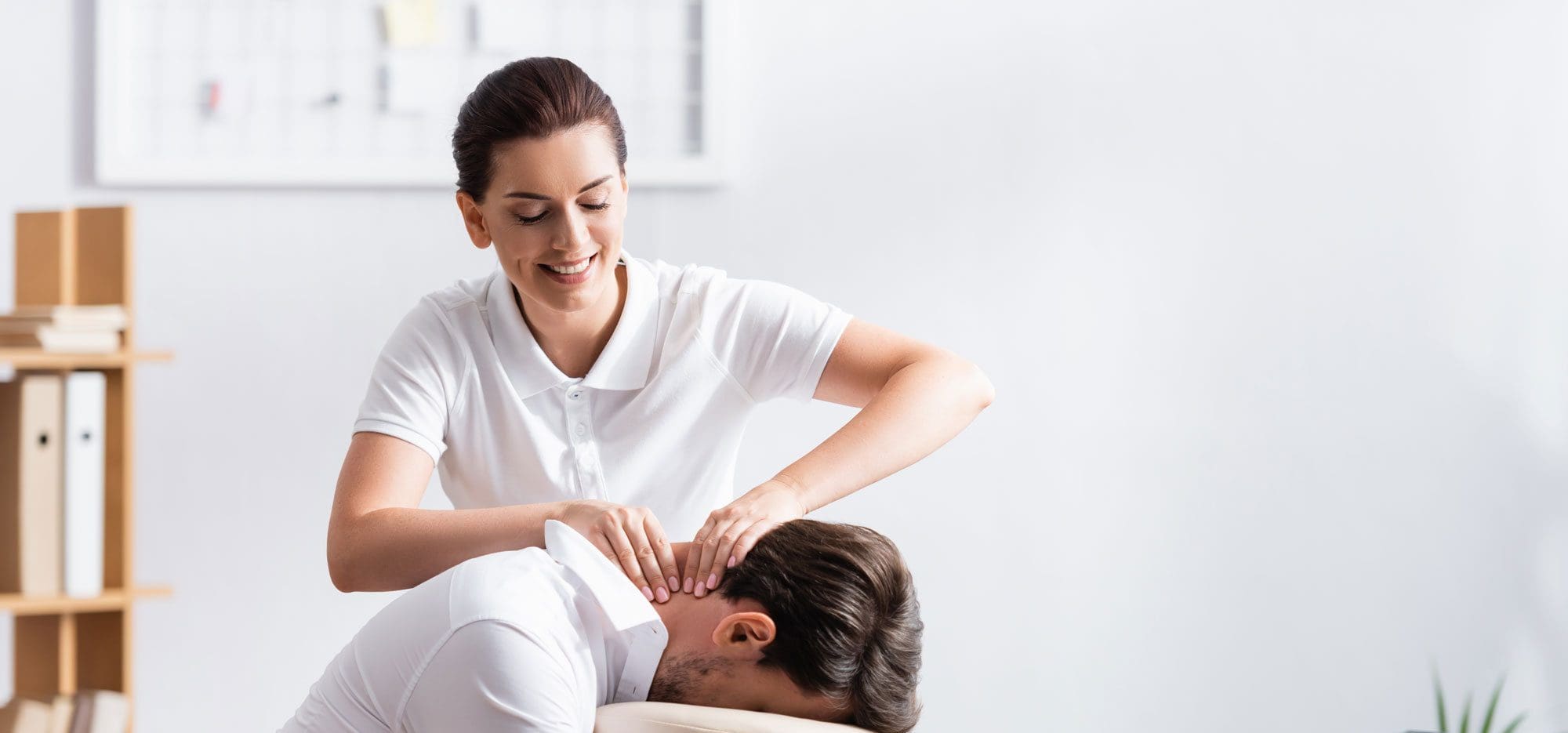The image features a detailed, serene setting where a woman is seen massaging a man's neck. The man, positioned slightly to the left and facing down, has brown hair and is wearing a white shirt. His posture suggests he is relaxed, allowing the woman to focus on his neck. She, wearing a white polo shirt and pink nail polish, is centered in the image slightly to the left and can be seen chest-up, smiling as she works intently on the man's neck muscles. The background is predominantly white and includes the back wall, a partially visible picture hanging on the top left, and some storage drawers or dressers in brown and light brown tones on the bottom left. The setting overall conveys a professional yet calming atmosphere typical of a massage therapy room.